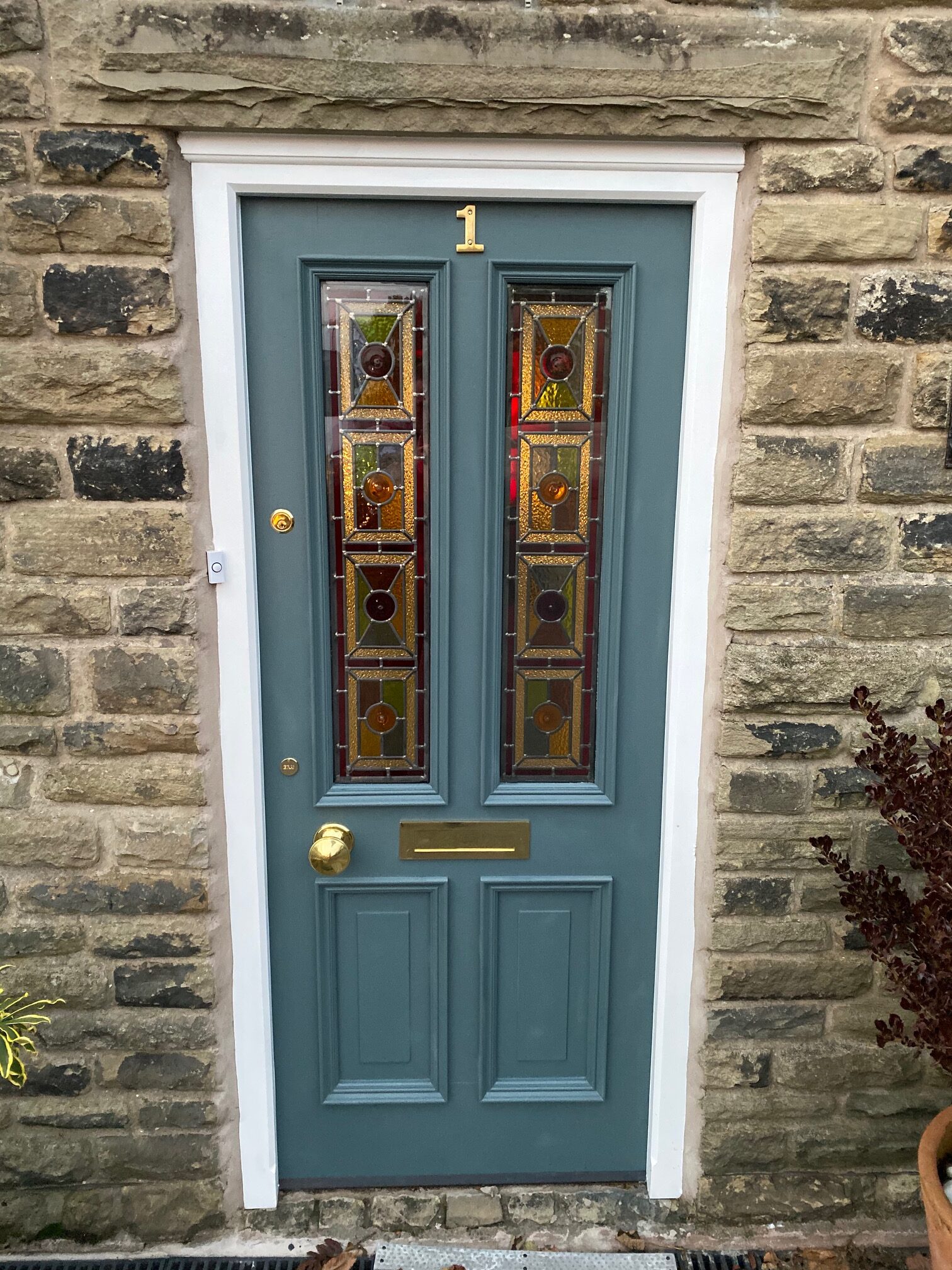The image depicts a door situated in the center of a tan-colored brick or gray stone building. The door is a darker shade of blue, resembling a bluish-green or darker robin's egg blue. It features a golden number "1" at the top, indicating the address. The door is adorned with several gold-colored elements, including a doorknob on the left side, a mail slot below it, and two key lock areas on the upper left. The door also has two rectangular stained glass windows, each divided into four sections, displaying a mosaic of colors like reds, greens, oranges, blues, and a bit of gold. The door is framed with a white structure, and a doorbell is positioned to the left. At the bottom right corner, a pot with flowers adds a touch of nature to the setting. Additionally, there are two plants on either side of the door, one with green leaves and the other with dark maroon leaves, which are slightly out of the main frame.